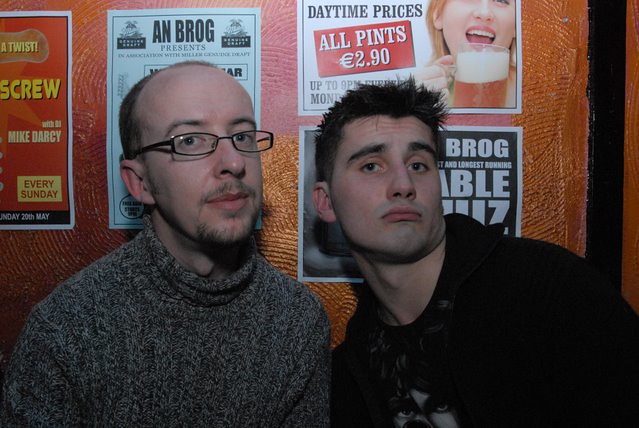In this color photograph, two men are posing in front of a wood-paneled wall adorned with various band posters and a prominent poster showing a woman holding a pint glass, advertising daytime prices for beer, with a text box indicating "all pints two pounds 90 pence." The scene appears to be set in a bar, likely located in London, as suggested by the details on the poster.

Both men are looking directly at the camera, with the photograph taken in landscape orientation. The man on the left features a receding hairline, is balding, and wears small wire-frame glasses. He sports a brown mustache and goatee and is dressed in a charcoal-colored, turtleneck sweater. His companion, on the right, has dark, spiked hair and is making a playful, exaggerated face while craning his neck towards the other man. He is outfitted in a dark coat and shirt.

The background wall has a distinctive texture resembling the decorative scrapes found in certain Buddhist monasteries, adding an interesting visual element to the otherwise dimly lit bar setting.